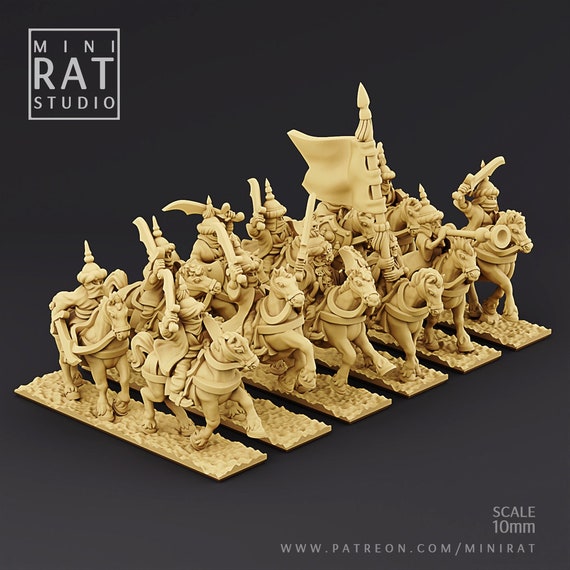The image features a sculpted art piece showcasing six intricately crafted clay figurines of Arabian horsemen. Each figure, mounted on horseback, depicts a dynamic scene with details such as a flag being raised and a horn being played, all set against a gradient gray background—light at the bottom and dark at the top. The figurines, light yellow in color, are presented on flat rectangular bases. In the top left corner, within a white-outlined box, the text "MINI RAT STUDIO" stands out in white, emphasizing "RAT." The bottom right corner notes the scale of the figures as 10mm with the URL "patreon.com/minirat" in white lettering.